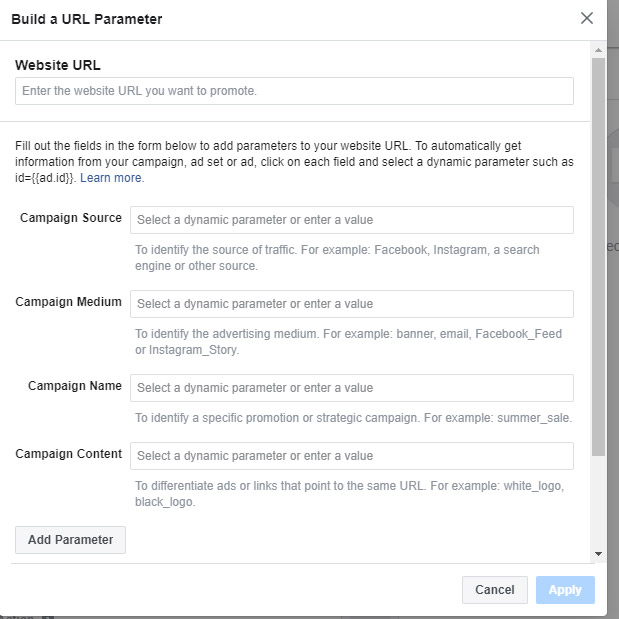The screenshot captures a cropped view of a form-like entry page from a website, titled "Build a URL Parameter." The window features a clean, white background with black text and grey text for form boxes and explanations. Highlighted by a scroll bar on the right, the top of the form includes an input field with a placeholder reading "Enter the website URL you want to promote." Below this, four more input fields are labeled for various parameters: CampaignSource, CampaignMedium, CampaignName, and CampaignContent. An "Add Parameter" button is positioned under these fields. At the bottom right corner, two prominent buttons are available: "Cancel" and "Apply."